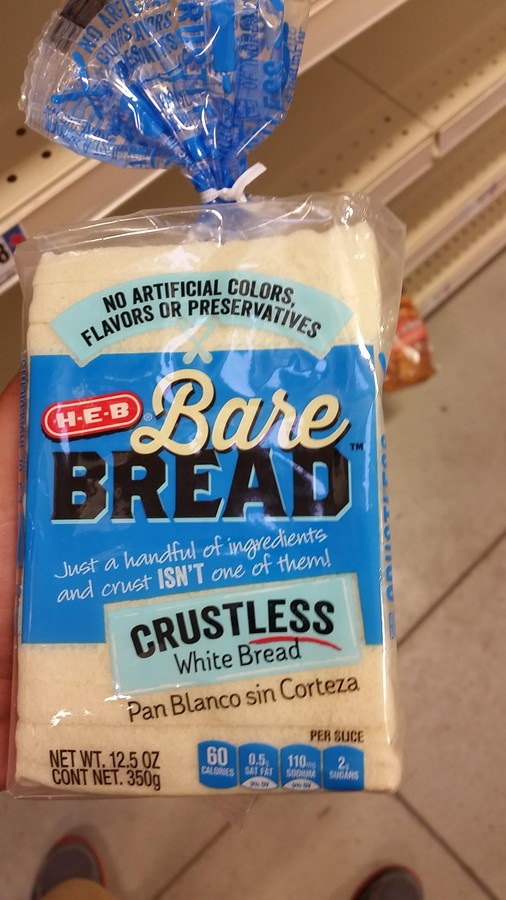The photograph showcases a product from a grocery store named Bare Bread, which appears to be produced by a company with Jewish origins, likely making it kosher. The bread is crustless, white, and marketed with the tagline, "Just a handful of ingredients, and crust isn't one of them." The packaging primarily consists of clear plastic, allowing a view of the bread inside, with light blue accents and bold black lettering stating "Bare Bread." Nutritional details are prominently displayed, indicating that each serving has 60 calories, 0.5 grams of fat, 110 milligrams of sodium, and 2 grams of sugar. The net weight of the loaf is 12.5 ounces. Notably, the photograph was taken in a grocery store, evidenced by the cream-colored metal shelves in the background. The person taking the picture is seen standing, with their brown moccasin-like shoes visible at the bottom of the frame.